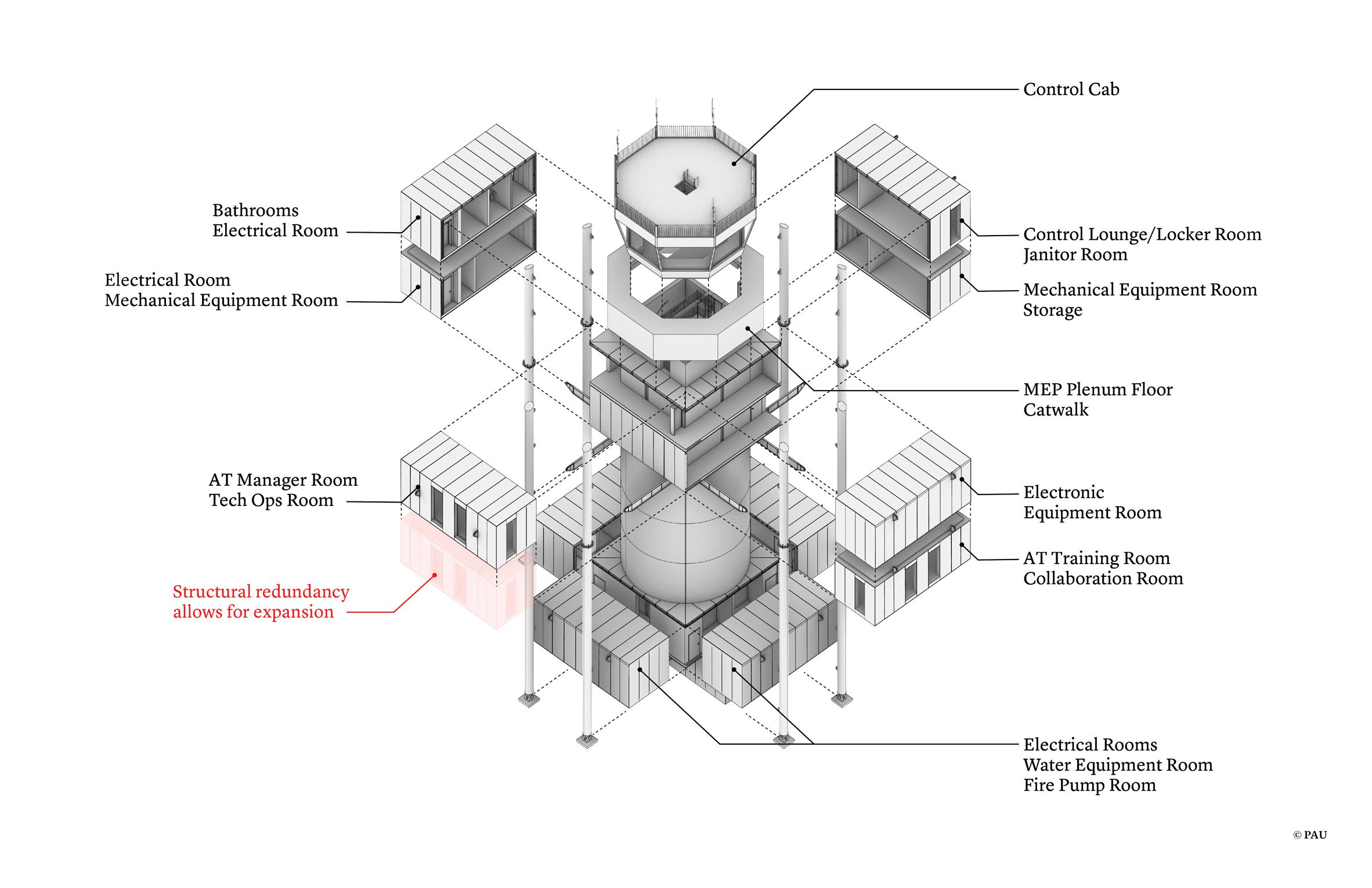This detailed black and white mechanical design diagram depicts a multi-level, rectangular, and octagonal building, with structural elements thoroughly labeled. The drawing is presented on a white background, highlighting various rooms along with their functions. For example, at the building's cylindrical core, the topmost section is labeled "control cab," surrounded by interconnected rectangular rooms such as bathrooms, electrical rooms, and an electronic equipment room. Further down, it features labeled sections like the AT manager room, mechanical equipment room, control lounge, locker room, janitor room, plenum floor catwalk, AT training room, collaboration room, and more. Notably, a distinct area in the lower left corner is highlighted in pink with red text reading "structural redundancy allows for expansion." This color contrast emphasizes this particular section within the otherwise monochromatic layout. The entire diagram methodically extends lines from each labeled part, demonstrating a comprehensive breakdown of the building or factory's structural and functional components.